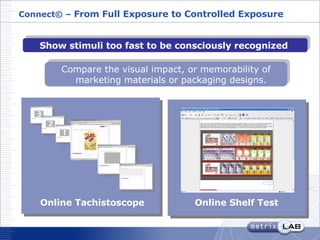The image is a low-resolution picture of a pamphlet featuring a detailed description of a marketing and testing tool. At the top left, it displays the word "Connect" followed by "from full exposure to controlled exposure." Below this, it reads "shows stimuli too fast to be consciously recognized" in dark blue with white letters. The next segment, in light blue, states, "compare the visual impact or memorability of marketing materials or packaging designs." The pamphlet visually demonstrates different aspects of the tool, including multiple open windows—six in total—one labeled "Online shelf test" with a blue background and white letters. At the bottom, the word "metrics" appears in blue followed by "lab" in white, set against a blue border. The background of the pamphlet is predominantly white, with sections showing various stimuli, suggesting the visual comparison capabilities of the system.